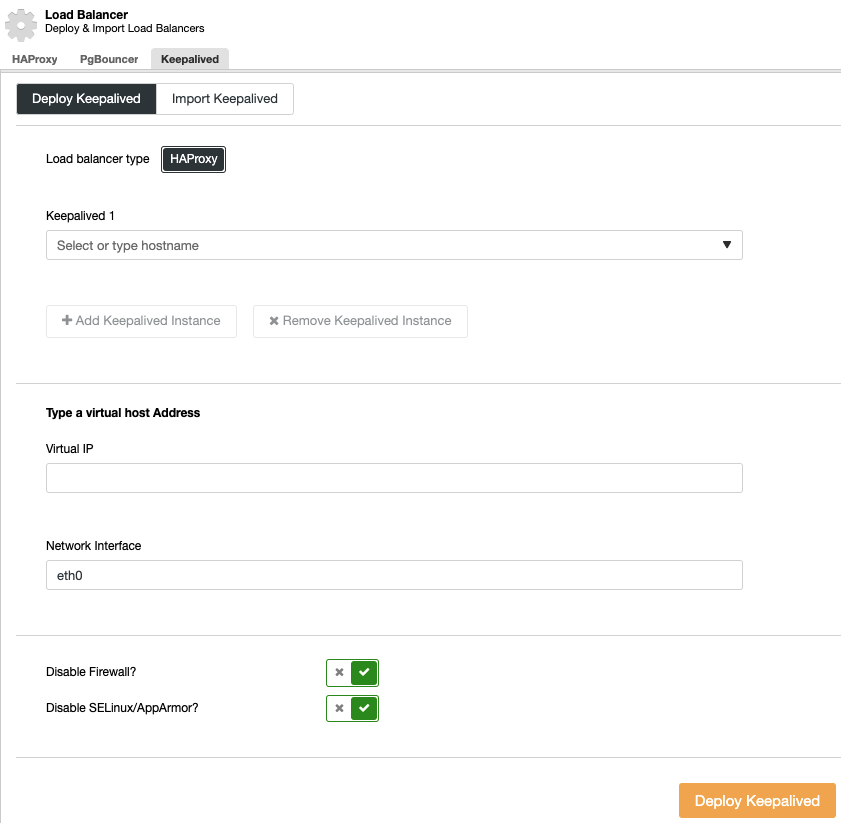The image is a screenshot from a website with a clean, white background. At the top, in bold black text, "Load Balancer" is prominently displayed, with the "L" and "B" capitalized. Adjacent to this, there is a light gray icon.

Below the "Load Balancer" heading, the text "Deploy and Import Load Balancers" is noted. Further down, "HAProxy" and "PG balancer" are mentioned in bold, with "HAProxy" (all uppercase) and "PG balancer" formatted as one word with a capital "P," lowercase "g," and capital "B".

The "Keepalived" load balancer option is highlighted next. The term "Keepalived" is fully capitalized. Moving down, there's a black background section with white text stating, "Deploy Keepalived," followed by an instruction to "Import Keepalived" on a white background.

Next, the "Load Balancer Type" is specified, with "HAProxy" in a black box and "Keepalived" mentioned below it. There’s a prompt to "Select or Type Host Name" accompanied by a dropdown menu. Additional options include "Add Keepalived Instance" and "Remove Keepalived Instance." 

The text "Type of Virtual Host Address" is in bold, followed by "Virtual IP." Below, "Network Interface" is specified as "eth0." At the bottom, options to "Disable Firewall" and "Disable SELinux/AppArmor" are listed.